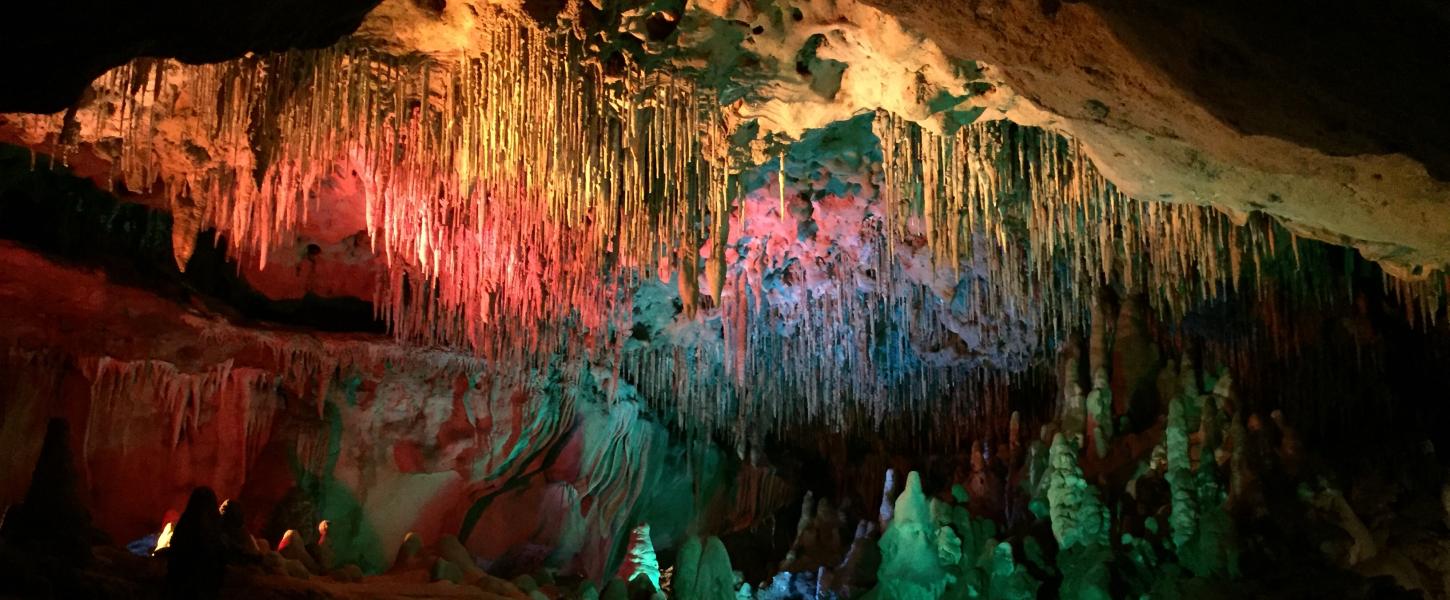This image captures the captivating interior of a large cave, highlighting a professionally photographed, horizontally rectangular landscape. The cave boasts an array of stalactites and stalagmites, with the stalactites resembling icicles hanging from the rugged, yellow stone ceiling, and the thicker stalagmites extending upward from the bumpy, rocky ground.

The scene is illuminated by strategically placed interior lighting, casting otherwise unseen colors and creating a vibrant tapestry throughout the cave. The top of the image is particularly expressive, dominated by a striking streak of yellow rock. Intermixed are hues of pink, aqua, green, and light green, contributing to an ethereal atmosphere. These colors transition and blend, with yellow, purple, and blue-red hues clearly discernible amid the formations. The intricately lit cave not only highlights the natural structure but enriches the visual experience with its chromatic diversity, creating a mesmerizing and unforgettable scene.